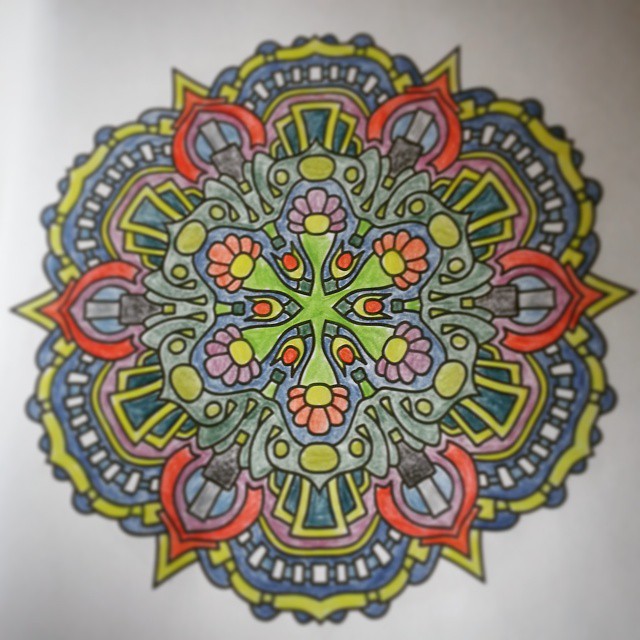This detailed photo showcases a page from a coloring book, featuring an elaborate Mandala design that resembles an intricate, flower-like pattern. The central part of the image is sharply focused, while the edges show a slight blur, drawing attention inward. The background is a crisp white, providing a stark contrast to the vibrant array of colors adorning the Mandala. Meticulously filled in with pencil crayons, the design bursts with shades of yellow, blue, green, purple, red, pink, as well as black and white accents. The coloring is precise, with no marks outside the lines, emphasizing the skill and care taken by the artist. There are no figures or text present, and the setting remains ambiguous, allowing the viewer to solely appreciate the artistic detail and colorful execution of the Mandala design.